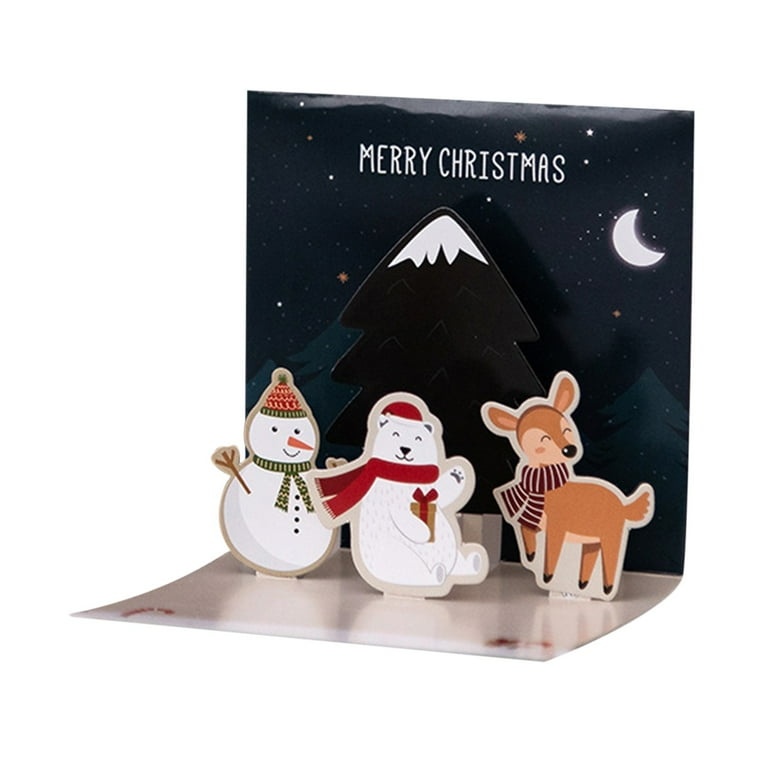This image depicts a pop-out Christmas card set against a starry night sky with a crescent moon in the top right corner. The foreground features three animated characters evenly spaced: a snowman on the left, a polar bear in the center, and a reindeer on the right. The snowman wears a green scarf and a knitted green and red cap, with a carrot nose and stick arms. The polar bear, positioned in the middle, dons a red scarf and cap while holding a gift. Behind the polar bear is a black Christmas tree with a white, snow-capped top. The reindeer on the right is brown, without antlers, and has a dark brown and white scarf. Above these characters, "Merry Christmas" is written in white text, completing the festive scene.